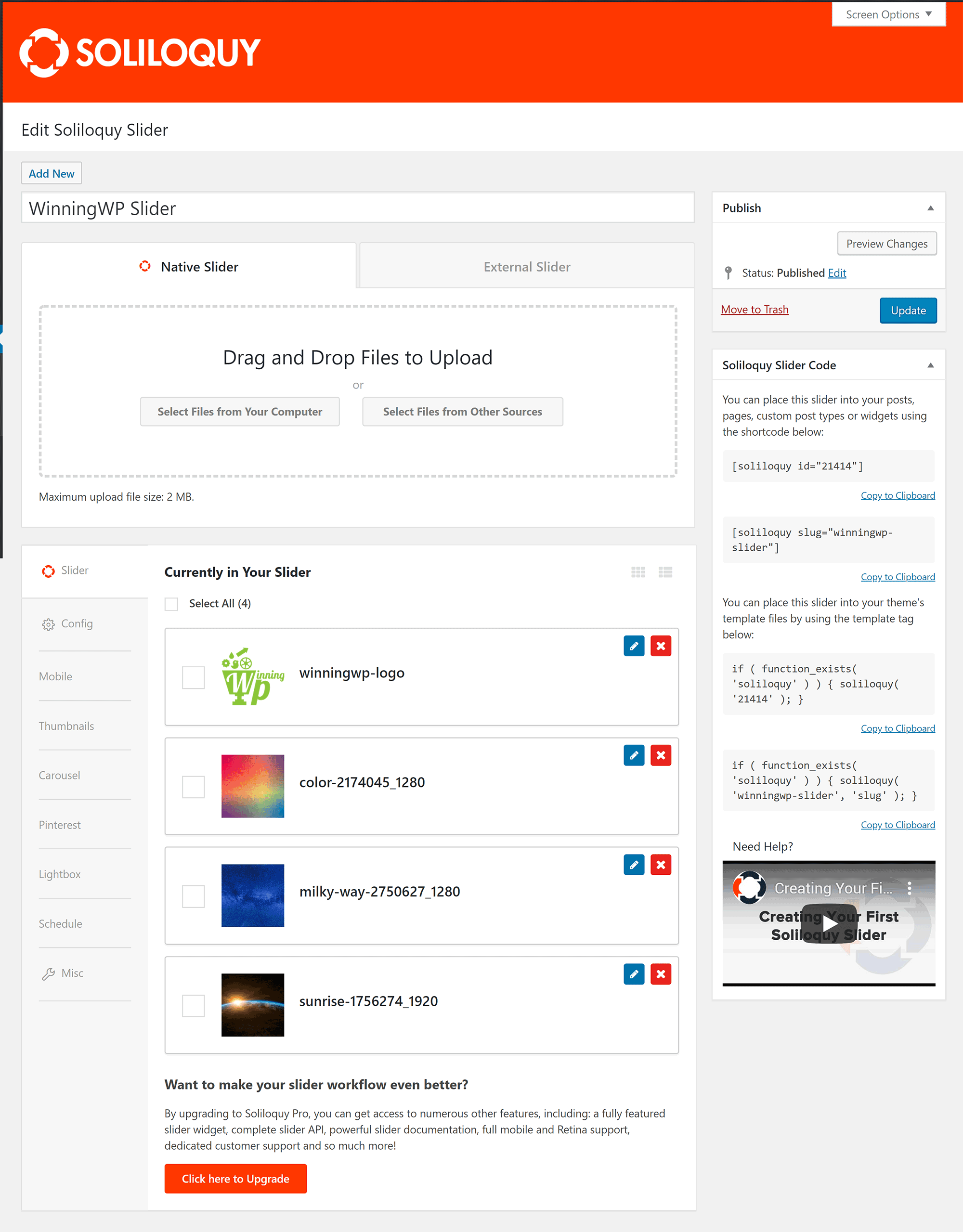The image features a user interface with a predominant red border at the top that spells out "SOLILOQUY" alongside a small, blurry, roundish logo. Below this red header, there's a white box bearing the text "Edit SOLILOQUY Slider," which stands out clearly against its background. The main section of the interface has a light gray background with a prominently placed text box at the top that reads "Winning WP Slider." Directly below this text box, there are several labeled sections, one of which is "External Slider." The clarity of some text in this area varies. Additionally, there's a specific area prompting users to "Drag and Drop Files to Upload." Underneath this section, there are two light gray-colored buttons. The left side of the interface houses a vertical column, whereas the right side features a video at the bottom that appears clickable for playback.